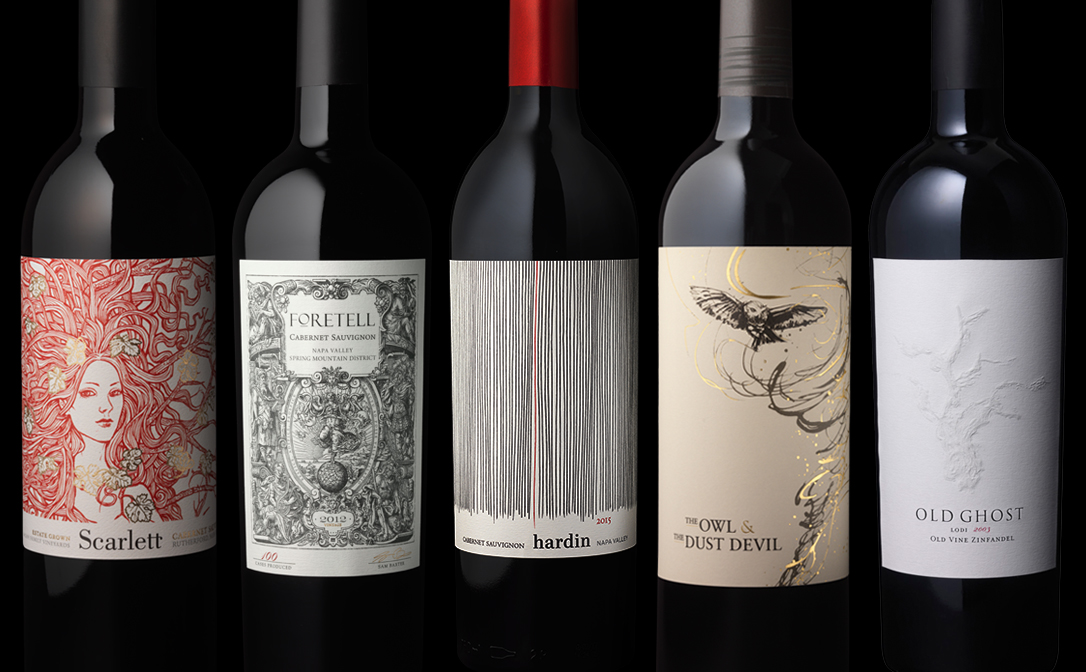The image showcases five distinct wine bottles set against a stark black background, highlighting their dramatic and gothic designs. From left to right:

1. The first bottle, "Scarlet," features an intricate label depicting a sketch of a female face framed by flowing, red-hued hair interwoven with green, black, and yellow flowers. The elegant label, coupled with the bottle's dark complexion and black cap, exudes a romantic and mysterious aura.

2. Next, the "Fortel" Cabernet Sauvignon hails from Napa Valley's Spring Mountain District. Its black bottle and cap are adorned with a white label bearing an elaborate black design that hints at a vintage garden statue motif, though the detail remains enigmatic.

3. The central bottle, "Hardin," boasts a strikingly modern label design. The white background is slashed by numerous vertical black stripes, with a single red stripe dramatically cutting through the center. This Napa Valley 2015 Cabernet Sauvignon further stands out with its red-topped cap.

4. "The Owl and the Dust Devil" bottle presents an enchanting scene on its beige label accented with gold and dark brown swirls, depicting a dust devil twisting upward with an owl in flight near the top. The bottle also features a unique brownish-black top, contributing to its ethereal and somewhat whimsical design.

5. The final bottle in the lineup, "Old Ghost," is an Old Vine Zinfandel from Lodi, 2003. Its pristine white label, embossed with a spectral design evoking smoke or a ghostly apparition, contrasts sharply with the bottle's black body and cap, creating a visually arresting effect.

The arrangement and lighting in the photo bring out the contrasting elements of these bottles, emphasizing their unique artistic labels and the shadowy allure of their dark glass forms.